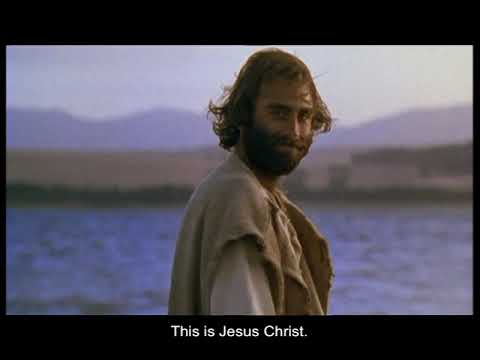A bearded man with long, slightly disheveled brown hair is posing for the camera, wearing historically inspired attire. His outfit consists of three layers: a white undershirt, a cream-colored shirt, and a sleeveless tan or yellow-tinted cloak on top. He stands near a large, blurry body of water, possibly a river or lake, with an out-of-focus one-story building on the far shore. Behind him stretches a distant mountain range, with a clear blue sky occupying the upper fifth of the image. His right shoulder is slightly closer, and his head is turned down and to the right. Text at the bottom reads, "opinions differ." The scene has a cinematic quality, suggesting it might be from a movie or a book, and the overall framing adds to this effect.